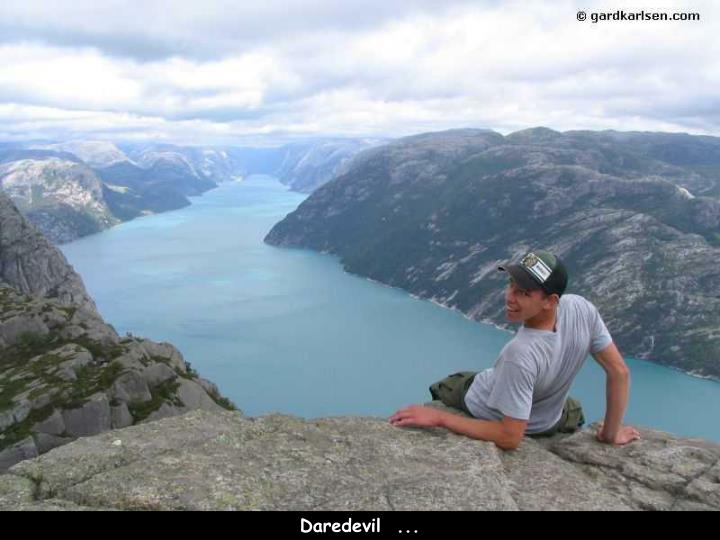In this detailed image, a young man with medium-colored skin sits daringly on the edge of a steep canyon cliff, gazing down into a ravine beneath a cloud-filled sky. He sports a green and black ball cap, a gray t-shirt, and green khaki pants. The sky occupies about a fourth of the image, overcast with multiple shades of gray and white clouds, leaving no clear skies visible. The central landscape features a striking blue river that zigzags through the middle of the image, flanked by imposing cliffs and mountaintops on either side. The man is positioned in the bottom right corner, his back to the photographer but his face turned around, appearing to smile. At the bottom of the picture, a black bar serves as a caption space, displaying the word "daredevil..." in white text. There is also a faint watermark at the top of the image that reads "copyright guard carlson dot com." The overall color palette is dominated by blues, grays, blacks, and greens, contributing to a dramatic and adventurous atmosphere.